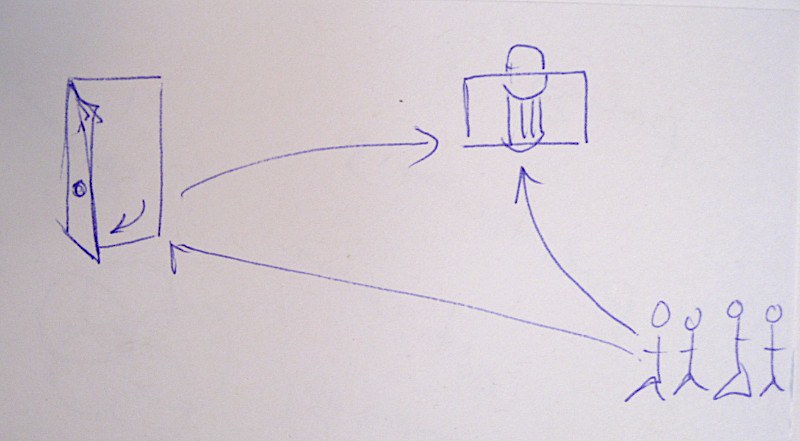This hand-drawn image features four stick figures rendered with simple, rudimentary shapes. Their heads are crudely sketched, and their arms appear as single straight lines extending from their bodies. Their legs are represented by arrows, creating a triangular shape at the lower part of their figures. Uniquely, one of the figures is entirely drawn as a triangle.

In the lower right-hand corner of the drawing, there is a depiction of a door. The door is portrayed in a very simplistic and messy manner, with a circular shape on its surface that likely represents a doorknob. An arrow is sketched to indicate the direction in which the door opens. This door is illustrated within a rectangular outline, representing the door frame.

Additionally, there is another arrow, also drawn messily, leading to a rectangular box. This box has a round circle intersecting its top edge, resembling a half-moon. This design is not elaborately detailed and its shape is notably a rectangle rather than a square.

A long line connects this rectangular box back to the stick figures, suggesting possible directional movement for the figures either towards the door or the box. The entire sketch is drawn on a white piece of paper, maintaining a simplistic, raw aesthetic.